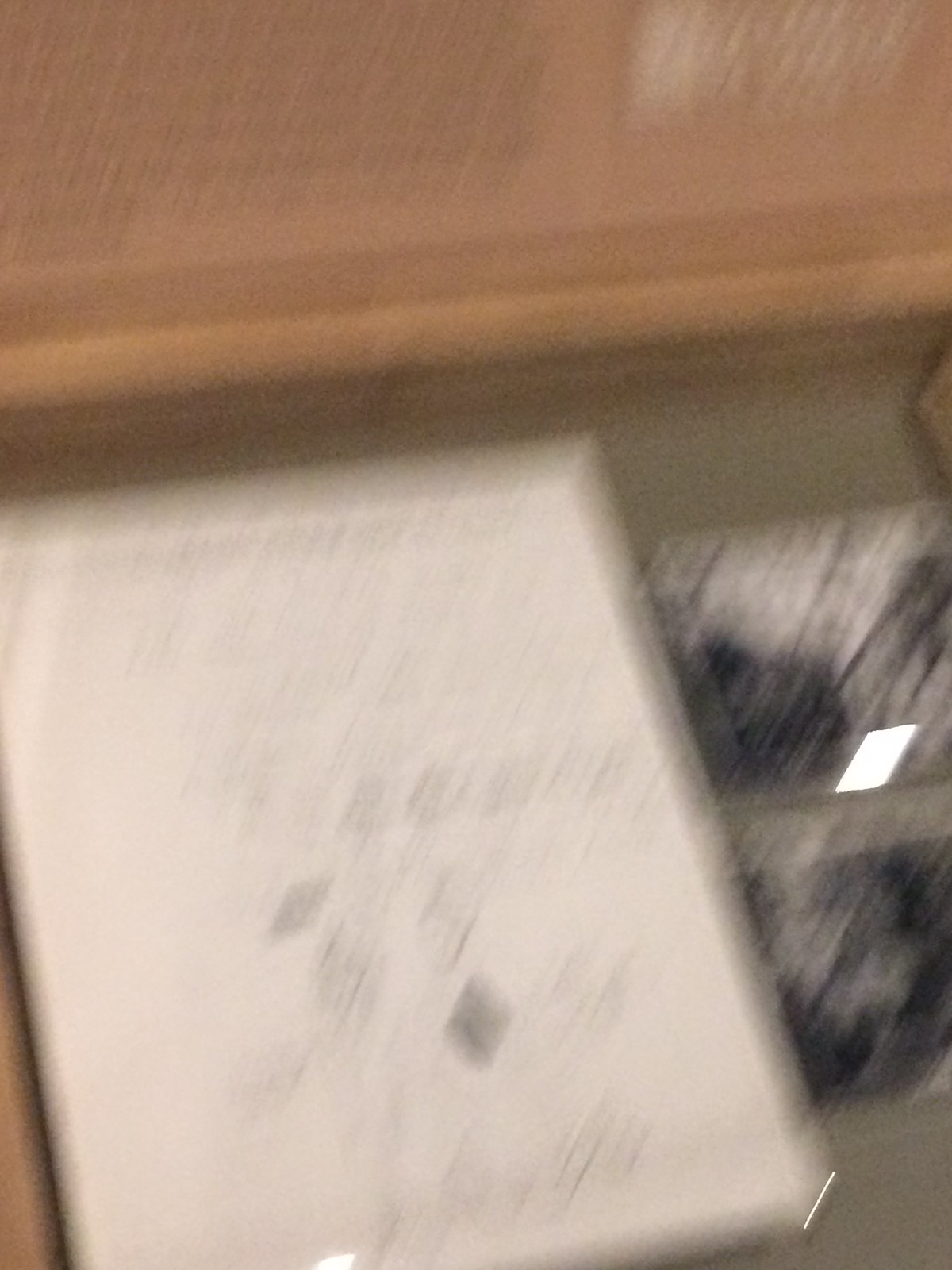The image depicts an extremely blurry indoor photograph taken at a slight angle, making it difficult to discern precise details. Dominating the upper quarter of the image, a brown-colored wooden area, possibly a cabinet or countertop, spans across, featuring a flat top with a subtle shelf or border beneath it. The right side of the photograph shows a reflective glass or window fragment with a distinct white appearance interspersed with black, catching a diamond-shaped light reflection. On the left side, a large white rectangular object, likely a sketch pad or book, occupies a significant portion of the image. The surface of this sketch pad reveals indistinct pencil drawings, including several diamond shapes centrally grouped, pointing in various directions. The graininess and out-of-focus nature of the photograph obscure further details, but a white rectangular glare in the center edge adds to the complexity of the visual elements.